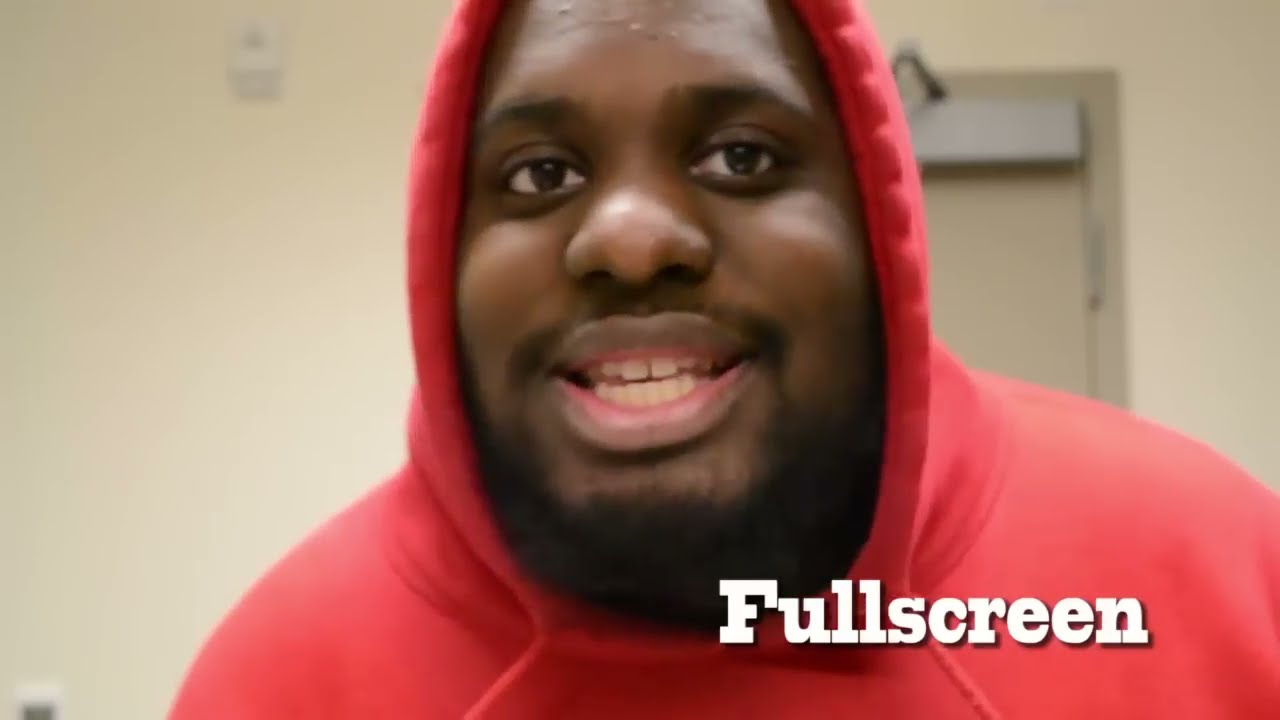This is a detailed close-up photograph of a black man wearing a red hoodie, which drapes over his shoulders. He has a full beard and mustache, with big brown eyes, and his mouth slightly open, revealing both his upper and lower teeth. There is a noticeable pink line along his bottom and upper lips. The man appears to be looking directly into the camera, which is positioned at about his chin height, approximately two feet away from him.

In the background, there is a light cream-colored wall adjacent to a brown door, which has a matching brown frame. Attached to the top left corner of the door is a silver metal door mechanism with a protruding arm, just behind the man's head. Additionally, on the wall's left side near the top, there is a two-toned box, white with a brown bottom, and in the bottom corner, another white square with a black square inside it. In the bottom right corner of the image, there is white text reading "fullscreen." The photograph, shaped like a high-definition TV screen, showcases a simple background that perhaps gives a faint hint of an industrial or commercial setting.